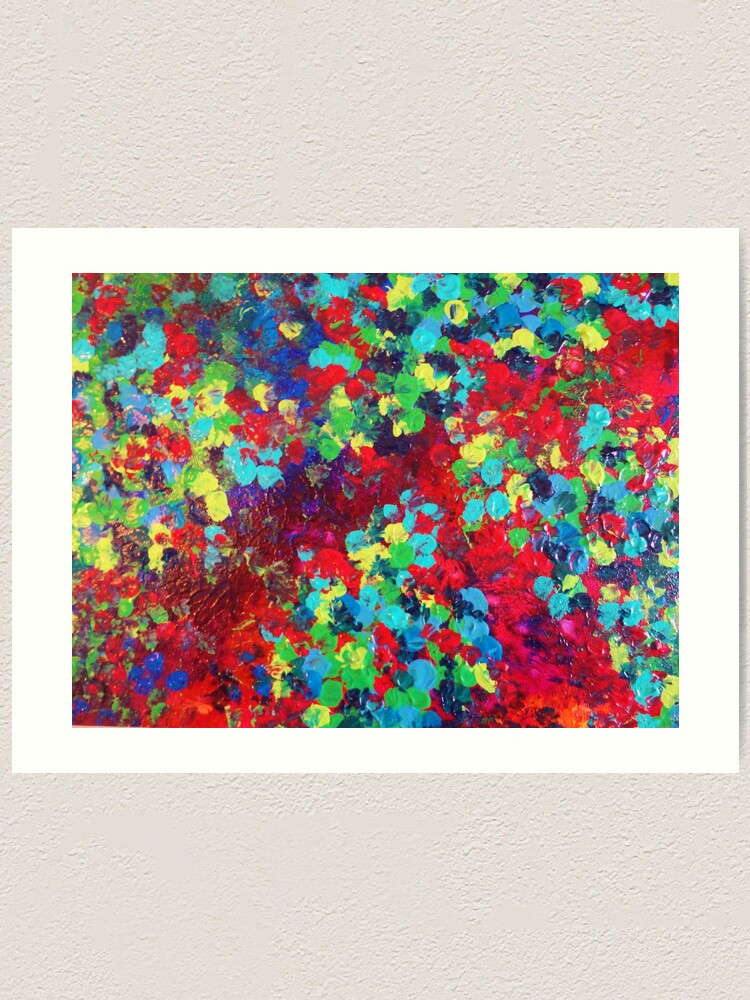The image depicts an abstract painting hanging on a cream-colored, rough and tactile wall with pockmarks. The painting has a nearly square shape with a white border. The artwork itself is a vibrant and dynamic composition of various colors, featuring an array of splotches and patches. Prominent colors include shades of blue—light blue at the top and dark blue at the bottom—along with teal, green, dark green, yellow, and red. In the center, there is a concentrated area of dark red splotches, while the right side features patches of black. The overall arrangement of colors appears random and abstract, creating a visually engaging and lively piece.